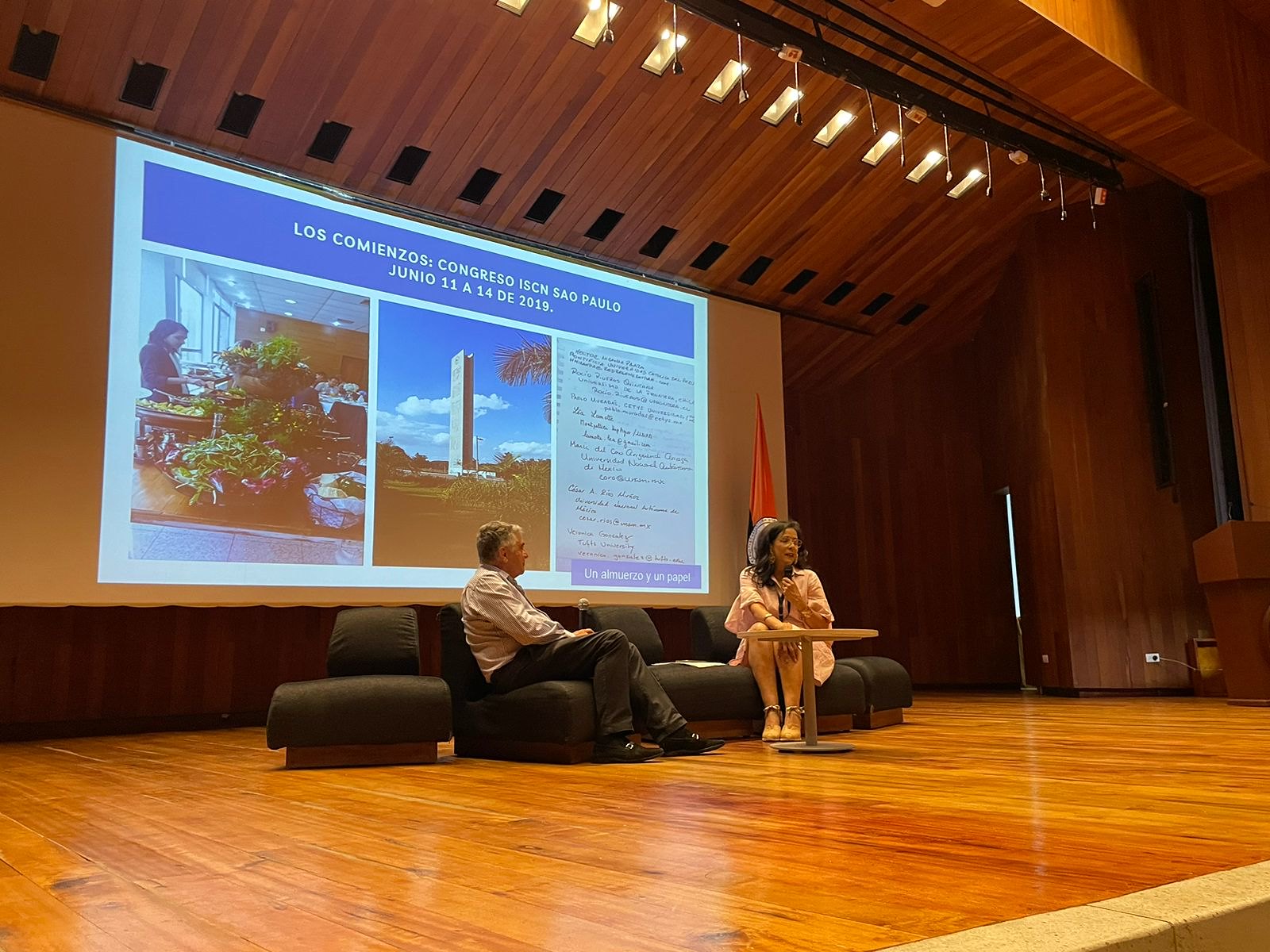The image captures a scene from a conference held on a stage made of shiny, golden-brown wooden boards. Two people are seated on what looks like a makeshift couch formed by arranging several gray recliners together. A man with short gray hair, dressed in gray slacks, black dress shoes, and a light blue collared shirt, is holding a microphone and looking towards a woman a few seats over. She has long black hair, glasses, and is wearing a pink dress. She also holds a microphone up to her mouth. In front of them, a small, plain round table with a silver pedestal stands on the stage. Behind them is a large projector screen displaying the text "Los Comienzos Congreso ISCN Sao Paulo Junio 11-14, 2019," along with images of some kind of tower and a woman surrounded by plants. A Brazilian flag flanks the screen, reinforcing the event's location and context.